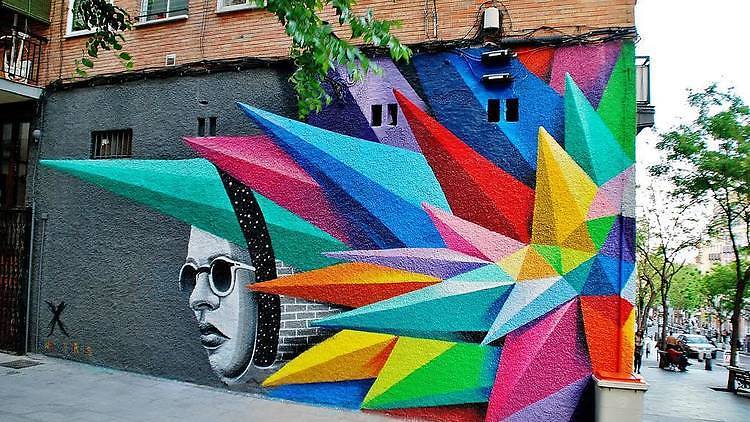This photograph captures a vibrant and dynamic mural on the side of a dark gray city building. The mural features an array of colorful, spiky geometric shapes, resembling multi-colored pyramids and crystals, in every hue of the rainbow, including purples, pinks, blues, yellows, greens, lavenders, teals, and oranges. These shapes create a striking, star-like pattern that surrounds a cylindrical form made to look like a gray brick tunnel. Emerging from this tunnel is the black-and-white profile of a person's face wearing dark sunglasses with white frames. The face, which appears somewhat androgynous and has full lips, gazes leftward with a stern expression. Additional elements in the mural include a black band with tiny dots around the face and a few tree branches. In the background, a busy city street with cars and pedestrian traffic is visible to the far right. The mural is signed with an 'X' and has some illegible writing below it, adding to the urban artistry vibe of the scene.